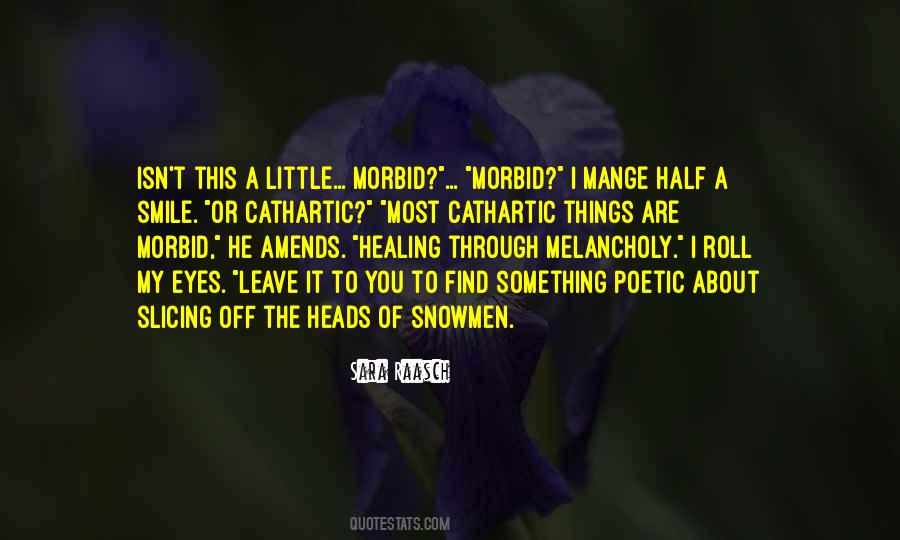In this image, a somber yet poetic quote stands out against a darkened backdrop featuring a purple-blue flower and splashes of green. The text reads: "ISN'T THIS A LITTLE MORBID, MORBID? I MANAGED HALF A SMILE OR CATHARTIC. MOST CATHARTIC THINGS ARE MORBID. HE AMENDS, 'HEALING THROUGH MELANCHOLY.' I ROLL MY EYES. 'I LEAVE IT TO YOU TO FIND SOMETHING POETIC ABOUT SLICING OFF THE HEADS OF SNOWMEN.'" Beneath the quote, in smaller white text, it reads "Sarah Rasch quotes at a.com." The image has a professional quality and is likely sourced from a quote or meme website, emphasizing the introspective and melancholic nature of the words.